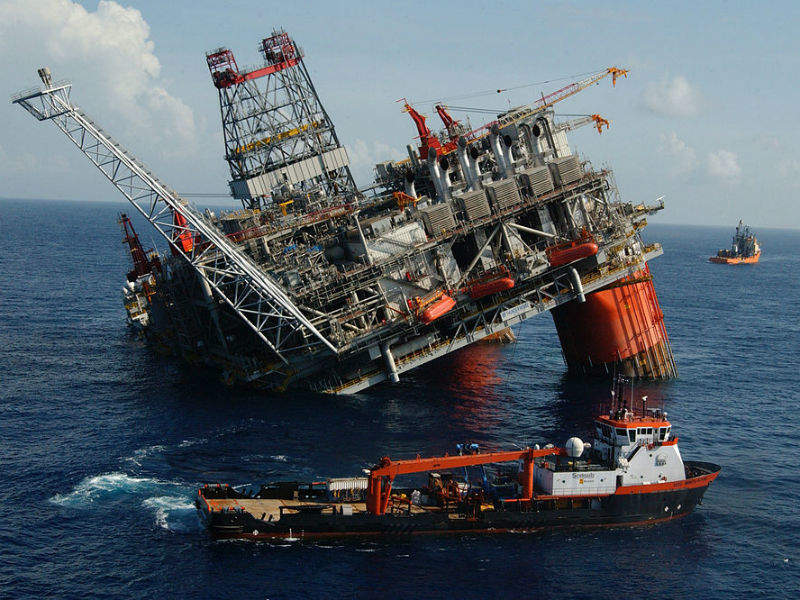In this captivating daytime scene dominated by blue skies with a few wispy clouds, we see an image of a partially sunken oil rig or barge in the middle of the ocean. The structure, which is a multi-floor complex made of steel and supported by large red and black metal cylinders, has experienced a severe accident. The left side appears to be compromised, with support beams missing and that part of the rig sinking into the water, causing it to lean heavily and precariously to the left. Numerous cranes and heavy machinery are visible atop the rig, adding to the complexity and industrial nature of the scene.

In the foreground of the image, a black, orange, and white ship, possibly a rescue or coast guard vessel, is positioned right in front of the distressed rig. To the right, another similarly colored ship, also perhaps a coast guard vessel, is present, suggesting an emergency response is underway. Additional boats, equally black with red and white hues, are seen navigating around the rig, indicating a coordinated effort to address the hazardous situation. The overall atmosphere of the image is one of urgent activity amidst the serene backdrop of the ocean and sky.